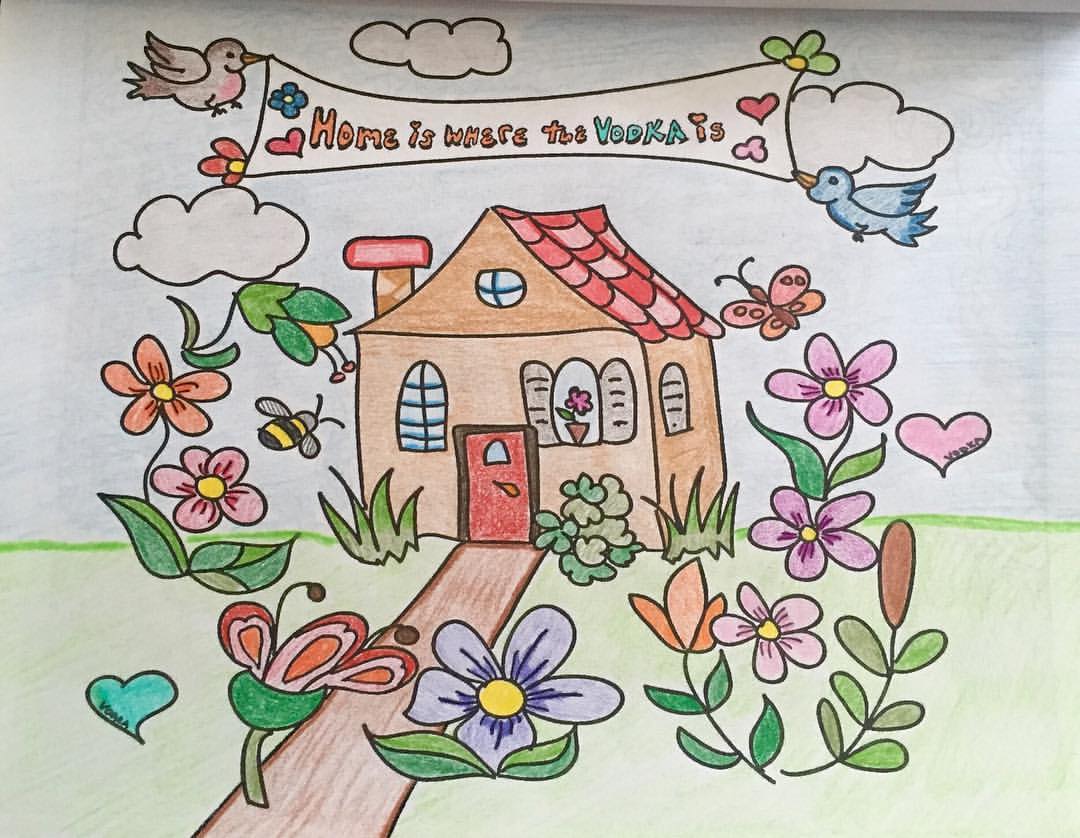This colored pencil illustration features a charming brown house with a red and white rooftop and gray shutters. The house boasts a circular window on the roof, a chimney with a red top, a red door, and open windows adorned with flower pots. A brown walkway runs across the lush green grass, which is dotted with flowers in vibrant shades of purple, orange, red, and pink, each having yellow centers. Above, the sky transitions from a slight blue to whitish hue, punctuated by fluffy white clouds. Two birds—one bluish-silver and the other brown with a rosy chest—hold a whimsical banner in their beaks that reads "Home is where the vodka is." The word "vodka" is highlighted in blue, while the rest of the text is orange. The banner is decorated with a flower and a red heart on one end, and a red heart and a pink piece of popcorn on the other. Additionally, a greenish heart with a bumblebee and a brown butterfly with a pink heart are found on either side of the scene, contributing to the overall playful and detailed aesthetic of the illustration.